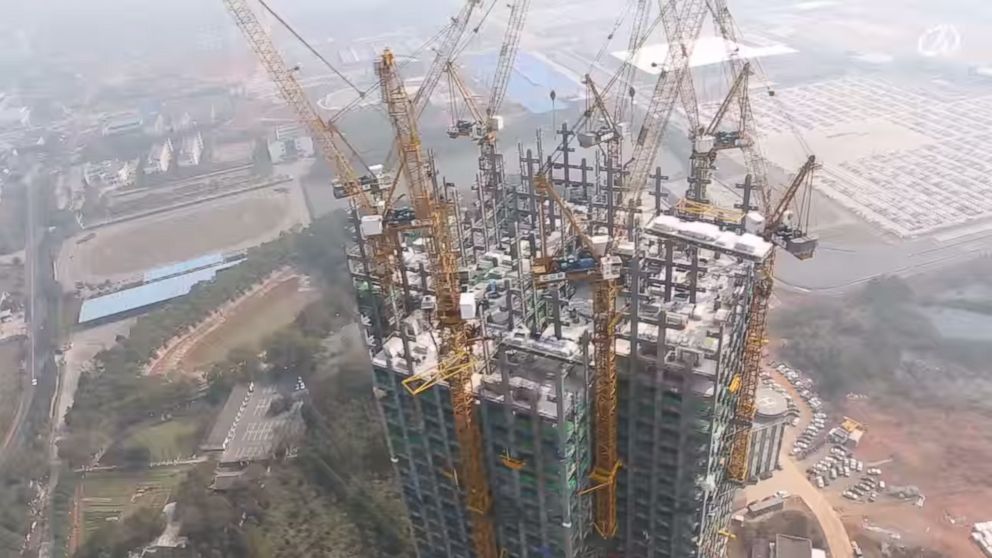This overhead view captures the detailed construction of a skyscraper, prominently positioned at the center of a landscape-oriented, color photograph. The high-rise tower, incomplete and under construction, boasts a unique architectural design with two intersecting rectangular shapes forming a corner facing the viewer. Rising vertically with squared, rectangular sides, the building features clearly defined layers and square window framings. Yellow cranes with long arms are stationed around the structure, actively working on erecting concrete pillars and additional levels, marked by visible rebar and scattered construction materials on the open top floor.

Surrounding the skyscraper, the ground below is a patchwork of brown dirt and green spaces. To the bottom right, a busy dirt parking lot is visible, while on the left side, there is an expansive outdoor space akin to a park with a field encircled by trees. This field transitions into a more rural landscape, where distant residential houses blend with vast green spaces and farmland, underscoring the semi-urban environment. The scene is enveloped by a gray mist, adding a subdued ambiance to the photographic realism captured by the drone.